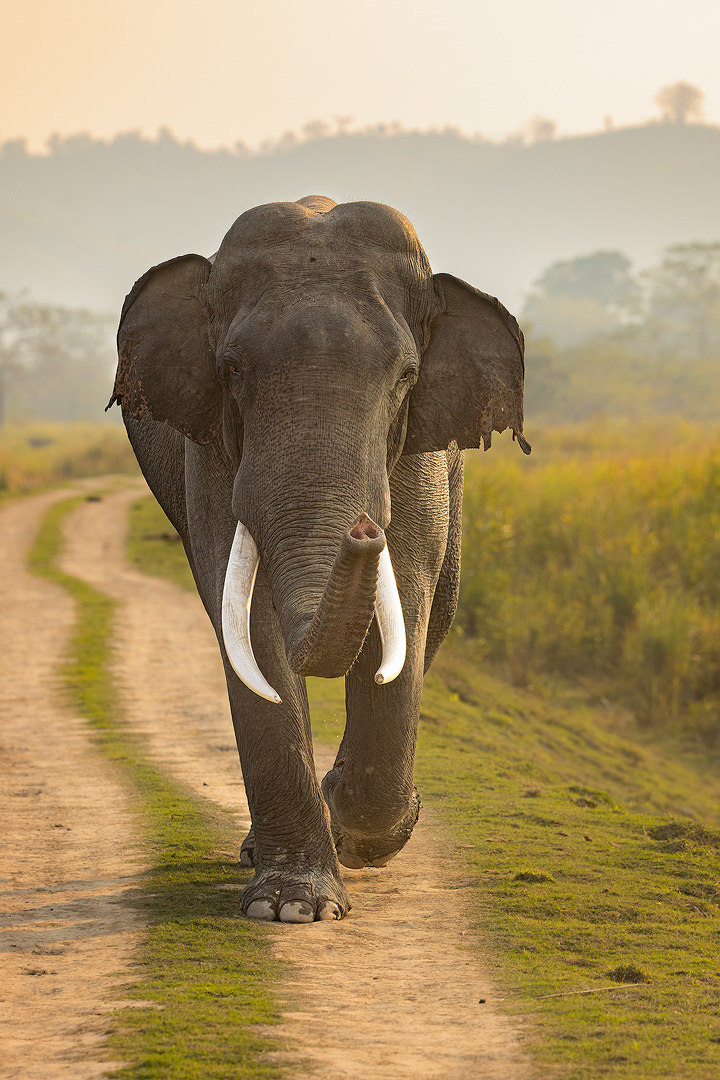This detailed color photograph, taken in portrait orientation, captures a majestic African elephant walking directly towards the camera along a two-lane dirt road. The elephant is massive, with imposing, curved white tusks protruding prominently from just below its raised trunk, which exposes its upward-pointing nostrils. Its large gray ears extend outwards, with the left ear noticeably tattered along the bottom edge, hinting at a history of adverse encounters.

The elephant’s right foot is firmly planted on the path, while its left foot is lifted mid-step, giving a sense of movement. A distinctive feature of the path is the strip of green grass growing in the middle, flanked by brown sand. Flanking the dirt road are patches of green and yellow grass, along with bushes.

In the background, the landscape reveals low hills or mountains shrouded in a foggy gray and white hue, with scattered trees visible through the mist. The sky has a mixed tone, with a tannish color on the left side blending into a whiter side on the right, indicating an overcast day. The photograph's style is photographic representational realism, capturing every detail with precision.